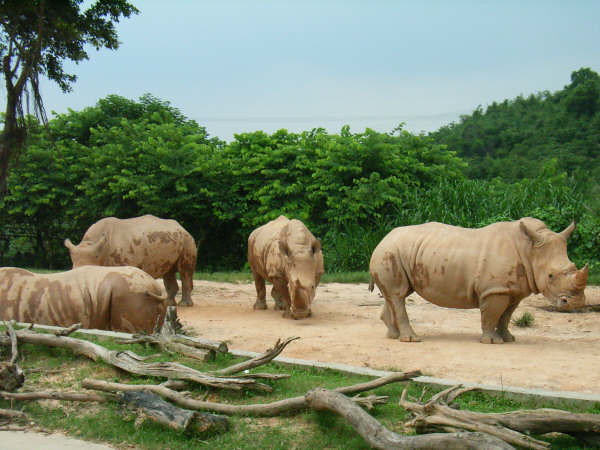In this vibrant photograph, four tan rhinoceroses stand prominently on a sandy dirt road surrounded by lush greenery. The two in front are clearly visible: one is positioned sideways while the other faces forward. A third rhinoceros, partially obscured, is turned away with only its back visible. A fourth rhinoceros stands at the far end. Each rhino is detailed with sharp horns on their nose, black beady eyes, and distinctive darker brown markings on their tough, tan skin. Their black feet contrast against the sandy ground, and they sport large funnel-shaped ears. Surrounding the path, thick brown fallen branches lie in a grassy area amidst a backdrop of dense, bushy green trees and tall grass. In the distance, tall hills with verdant foliage rise under a light blue, cloudless sky, suggesting a sunny day in this vibrant jungle setting.